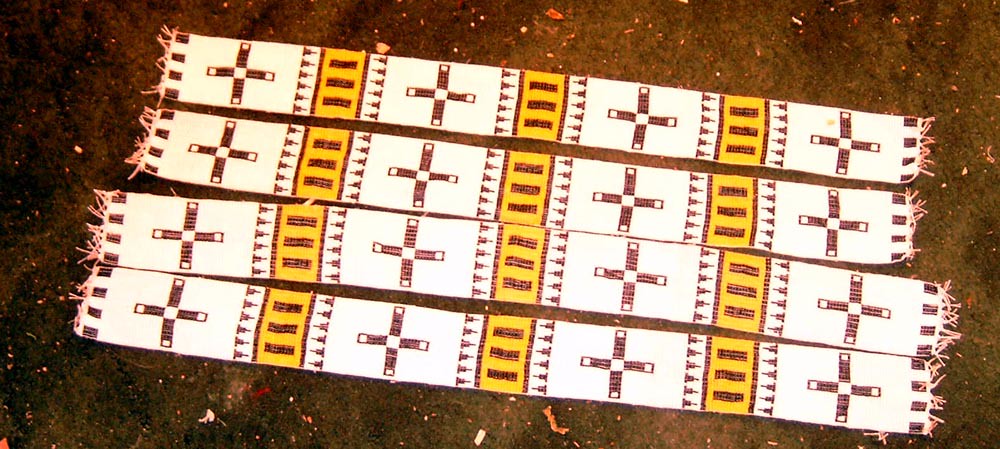This image showcases four rectangular banners, resembling ceremonial scarves, aligned parallel to each other. Each banner, adorned with little white tassels at both ends, features a repeating geometric design. The pattern consists of brown crosses with central and end white squares, flanked by yellow rectangles bordered with brown and containing three long brown stripes. Interspersed with these rectangles are white and brown triangles that add to the decorative motif. Notably, the two lower banners are slightly longer than the two upper ones, suggesting a possible distinction in use or wearer size. They are laid out on what appears to be a ground or rug strewn with litter, creating a stark contrast between the intricate, religious symbolism of the banners and their careless surroundings.